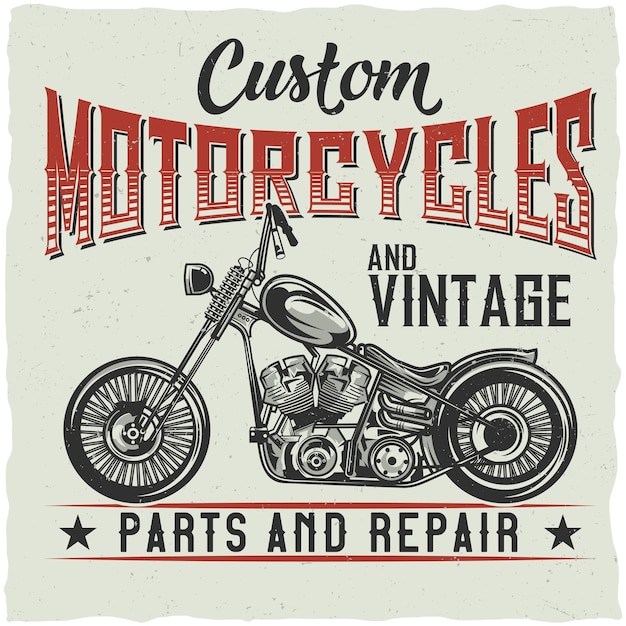The image features a cream-colored, square advertisement that seems to evoke a vintage feel with its irregularly torn edges and textured paper background. At the top, the word "Custom" is elegantly written in a cursive script in black. Just below, the word "Motorcycles" is prominently displayed in a bold, tattoo-like font that transitions from solid red at the top of the letters to horizontally striped red and white at the bottom. In the same distinctive font, the words "And Vintage" appear just beneath "Motorcycles." The center of the image showcases a stylized, screen-printed, grayscale motorcycle in profile, facing left. This motorcycle has high handlebars with visible springs near them, a prominent gas tank, and exposed engine components including motors, pipes, and belts. There is a low-angled seat with a small fender over the back wheel. The motorcycle appears to be positioned on a red band that stretches across the bottom of the ad. Below this band, with a star flanking either side, the words "Parts and Repair" are displayed in matching fancy typography. The entire advertisement exudes a sense of nostalgia and craftsmanship, combining detailed graphic elements with a carefully chosen color palette.